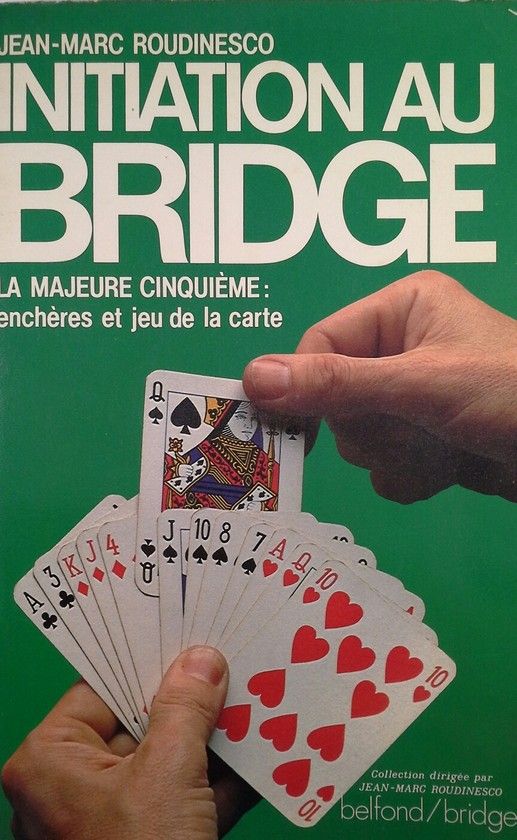The image depicts a portrait of a French book cover titled "Initiation au Bridge," written by Jean-Marc Roudinesco. The cover, dating perhaps from the 1970s or 80s, serves as an introduction to the card game Bridge. It features a photograph set against a green background showcasing a pair of hands, where the left hand is fanning out a Bridge hand sorted by suit. The cards displayed are the Ace of Clubs, Three of Clubs, King of Diamonds, Jack of Diamonds, Four of Diamonds, Queen of Spades (being pulled out by the right hand), Jack of Spades, Ten of Spades, Eight of Spades, Seven of Spades, Ace of Hearts, Queen of Hearts, and Ten of Hearts. The book also includes a subtitle, "La Majeure Cinquième, Enchères et Jeux de la Carte," which suggests a detailed focus on specific aspects of Bridge. In the bottom right corner, the text "Collection dirigée par Jean-Marc Roudinesco, Bellefonte/Bridge" indicates that this book is part of a series on card games under a particular publisher. All textual elements are rendered in white font over the green background.